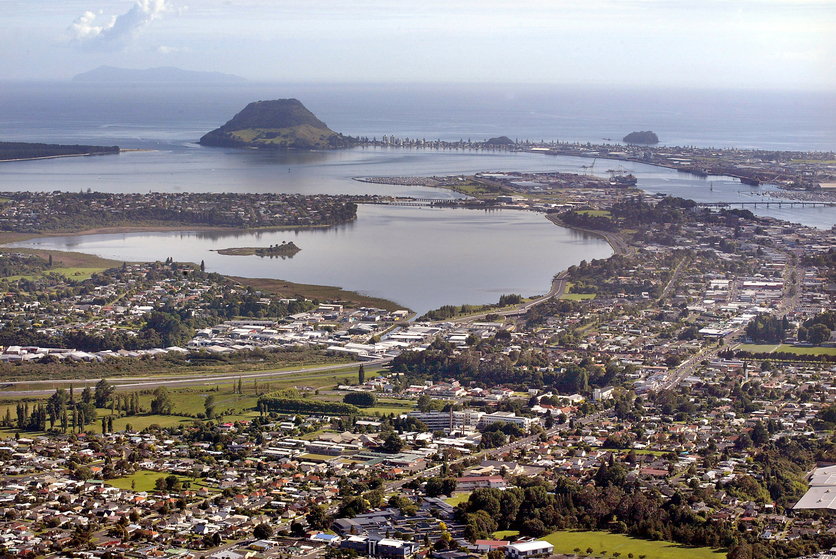This photograph captures an aerial view of a coastal city nestled between lush greenery and an expansive body of water. The community, dense with residences and buildings of varying sizes and colors, is situated along the coastline, adjacent to a serene bay that stretches inward before opening up to what appears to be the ocean. A prominent flattened volcanic hill sits in the middle, adding a distinct geological feature to the landscape. The bay features a small inland island or peninsula, with a road cutting through the town, lined with thick clusters of trees. Towards the far left, the bay becomes almost enclosed, resembling a cove, while in the distance, beyond a larger rock edifice, the vast open sea extends towards a hazy horizon, shrouded in an overcast sky. The scene is serene yet vibrant, juxtaposing the gray-toned sky with the green landscape and the colorful array of buildings.